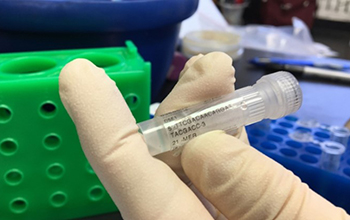A person is working in a medical or laboratory setting, focused on handling a plastic tube. The individual's left hand is gloved, using the thumb, index finger, and middle finger to hold the tube, which has a sticker with indistinct letters. The background features an array of greens and blues. Notably, a green test tube holder is visible alongside a blue test tube holder containing empty tubes with their tops removed. The scene is set on a table, dotted with indistinguishable writing utensils and miscellaneous plastic items. The image's palette includes white, various shades of blue, green, and the clear color of plastic. No additional text or images are present beyond the label on the plastic tube held by the gloved hand. The overall image is somewhat blurry, adding an element of indistinctness to the finer details.